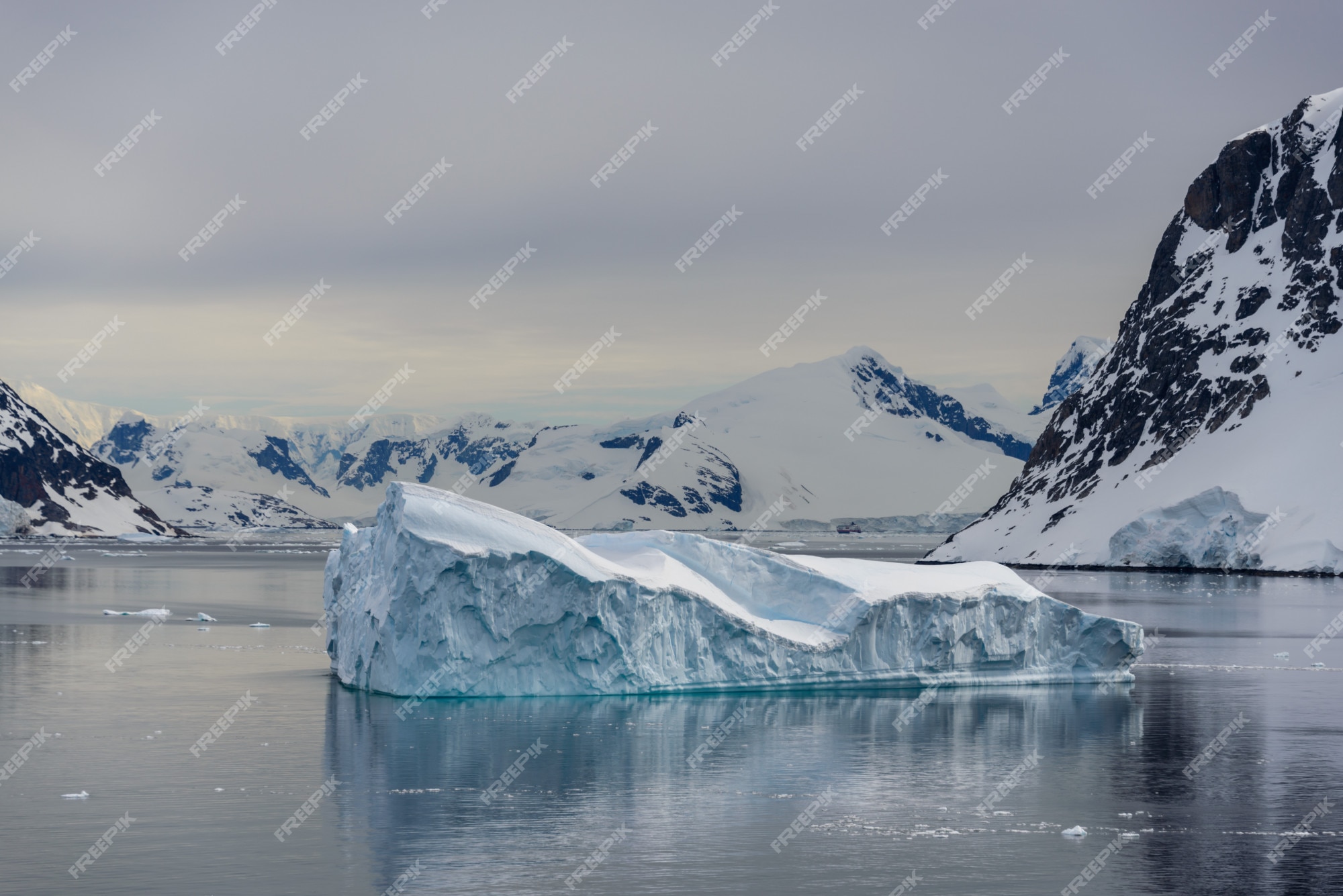This color photograph captures a moody, bluish-grey scene featuring a large iceberg floating in eerie, grey water. The iceberg, predominantly taller on its left side, has a jagged square shape with multiple levels of snow and ice, presenting a greyish-green hue at its base. The water reflects the fairly large iceberg, which angles up towards the left. Diagonal white watermarks, indicating "Free Picks," are uniformly spaced across the photo from the top left to the bottom right corner. The background reveals either snow-covered land or larger icebergs, along with a darker rock formation peeking from the middle to the top of the image, partially covered in snow. The overcast sky further intensifies the cold, gloomy atmosphere, hinting that the location might be near the North or South Pole, given the presence of icebergs and the intensely frigid environment.